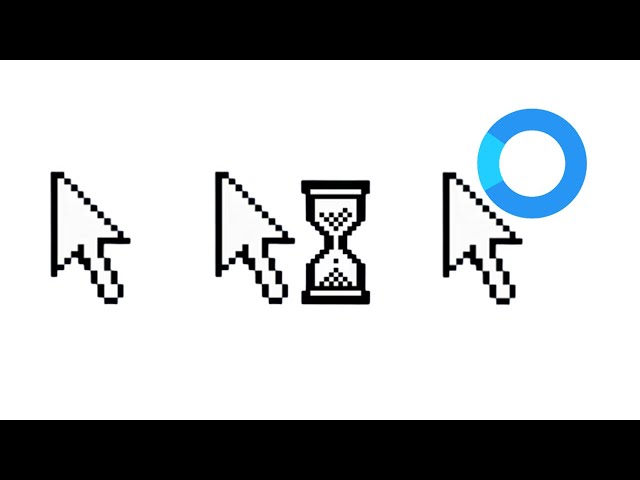The image showcases three distinct mouse cursor styles set against a pure white background, accentuated by black bars at the top and bottom reminiscent of a widescreen format. The leftmost cursor is a highly pixelated, traditional mouse pointer icon. The middle cursor, identical in style to the first, is accompanied by a pixelated hourglass to its right, indicating a wait state. The rightmost cursor features the same pointer with a light blue circular loading icon just above and to its right. The colors in the image consist primarily of black, white, and two tones of light blue in the circular icon. There is no text present, suggesting its use as a graphical representation, possibly for a video header or a digital screen indicator.